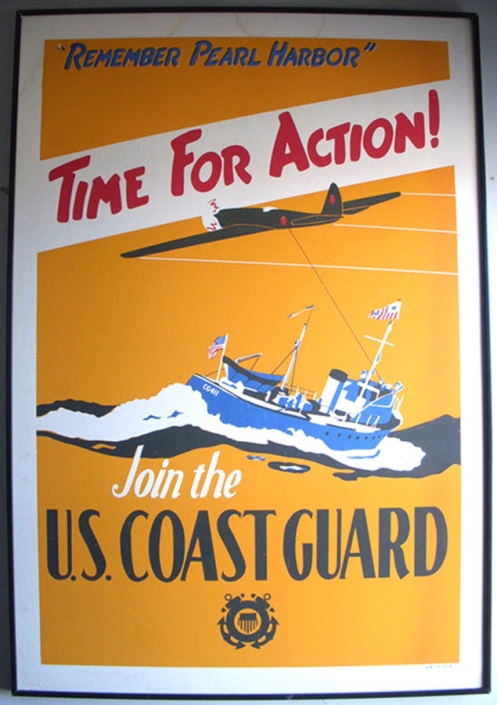The image is a rectangular World War II poster framed in a thin black frame with a white border. The central part of the poster has an orange background. At the top, in large blue capital letters, it reads "Remember Pearl Harbor." Below this, a diagonal white banner declares "Time for Action!" in red, bold letters. Just beneath the banner, a Japanese plane with red dots on its body and tail flies to the left. Below the plane, a U.S. Coast Guard ship battles through choppy waters, displaying the American flag prominently at the bow and other Allied flags. At the bottom, the text "Join the U.S. Coast Guard" appears, with "Join the" in white and "U.S. Coast Guard" in dark blue. The poster also features the Coast Guard seal, which is a circle with a small flag in the center, positioned below the text.